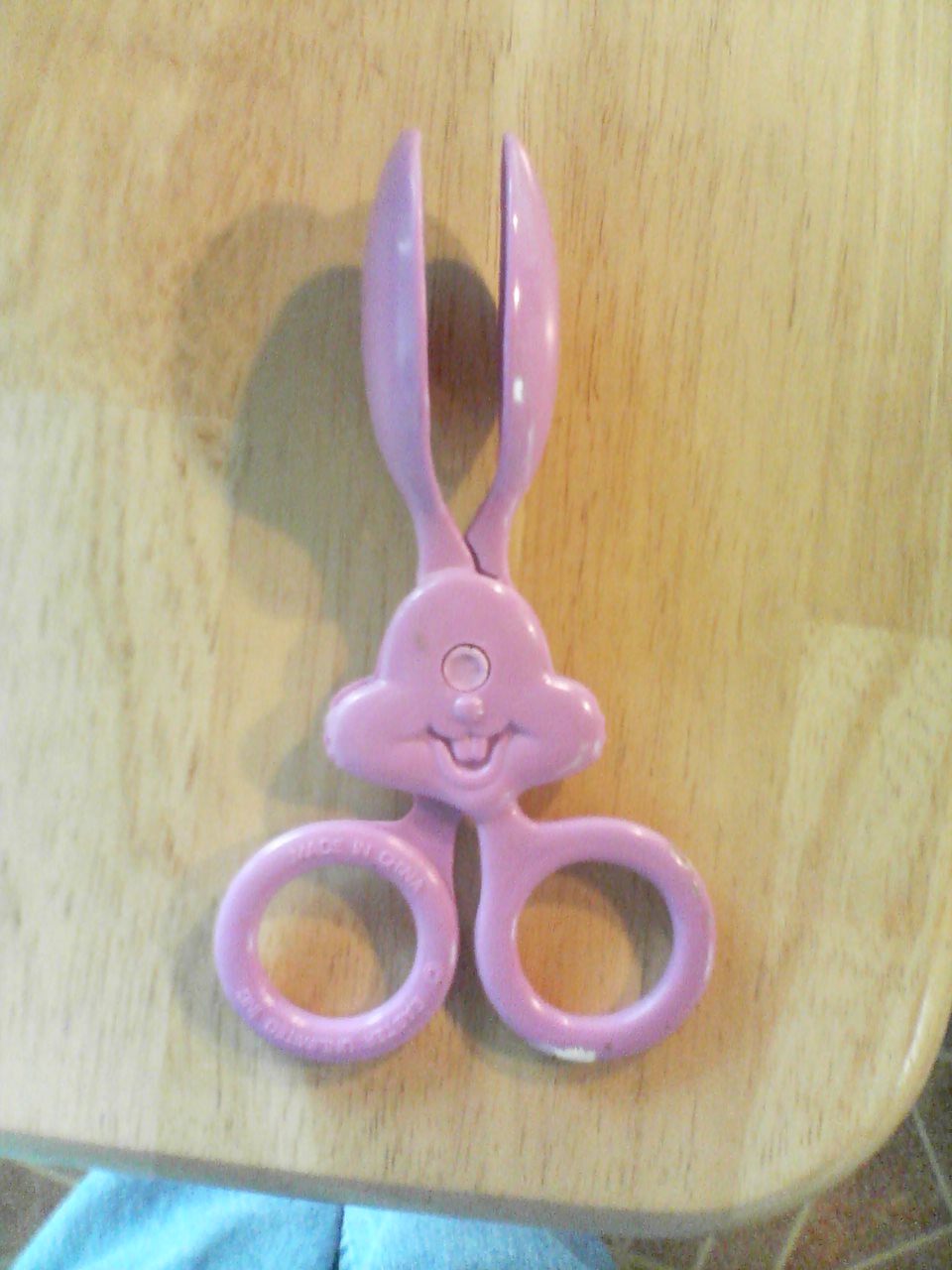In this color photograph taken from above, we see a pair of novelty children's scissors laid on a light brown wooden surface, possibly a school desk. The scissors are pink and designed with a whimsical bunny face in the middle. The bunny's face features a singular round eye, a nose, and a smiling mouth with a prominent protruding tooth, creating an endearing expression. The scissors' blades, facing upwards, resemble bunny ears. The handles are small and round, intended for a child's fingers. Strange shadows appear behind the scissors, including a peculiar balloon or light bulb-shaped shadow to the left. At the bottom of the image, there is a crumpled blue fabric, likely someone's pants, and to the right, part of a brownish surface with white lines, possibly tiling. The photograph seems to be of modest quality, suggesting it was taken with a cell phone or a similar device.